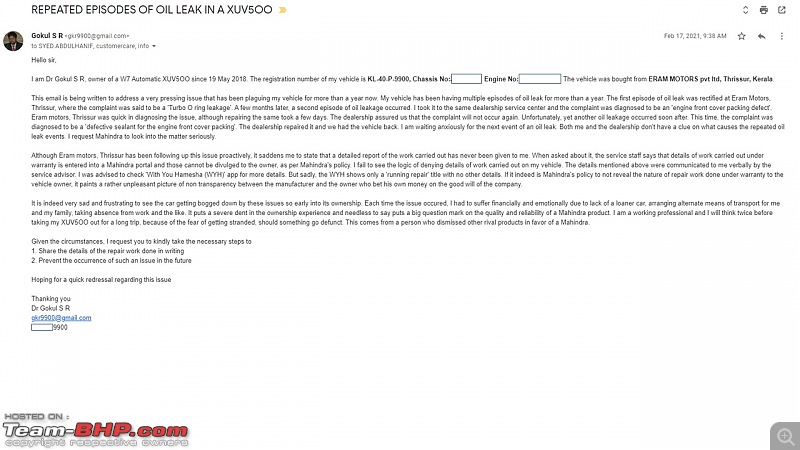Screenshot of an email regarding repeated episodes of oil leaks in an XUV 500. The email header reads "Repeated Episodes of Oil Leak in an XUV 500". The email is sent by Goku SR to customer care. Due to the small font size, the detailed content of the email is unreadable, but it appears to consist of three paragraphs, potentially discussing the issue of the oil leaks. The email is formatted with black text on a white background. In the lower left corner, there is a faint watermark that reads "Hosted on:" in gray font, followed by "team-bhp.com" in white and red font. Below this watermark is some additional unreadable gray text. Additionally, there is a small gray box in the lower left corner featuring a lighter gray magnifying glass icon with a plus sign in the center, which is commonly used to indicate a zoom function.